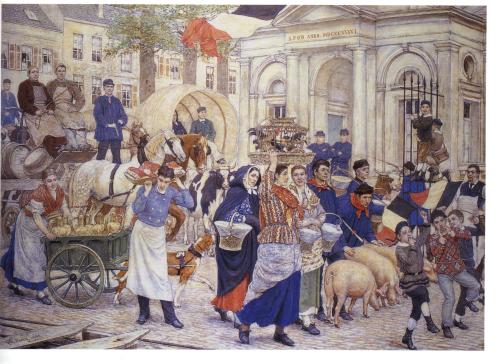This watercolor-style painting depicts a bustling outdoor market scene in front of a grand, cream-colored building with columns and arches. The scene is filled with a diverse array of people dressed in various shades of blue, with splashes of red and gray. On the left, a woman in a black robe carries a basket while another woman nearby balances a cage of chickens above her head. A man in a blue shirt and white apron carries something hefty on his shoulders, and behind him, a woman pushes a cart. A horse-drawn cart, driven by a standing man, carries two women dressed in aprons and brown shirts. 

In the background, residential buildings with multiple stories and windows rise up, framing the market scene. Near the bottom right corner of the image, a group of children interact or dance around some pigs, adding to the lively atmosphere. The ground beneath them is stony, typical of the pioneer days. Above the columns of the main building is some text, though it is too small to read clearly. The painting captures a snapshot of everyday life, brimming with activity and vibrant details.